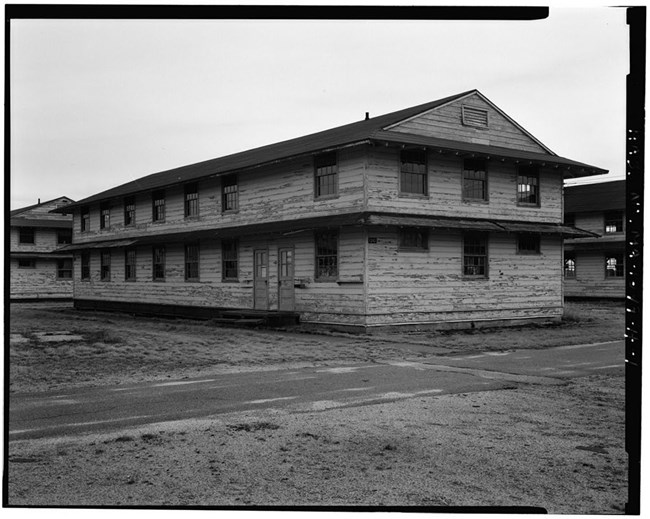This black and white photograph depicts a vintage, dreary scene of what appears to be an abandoned, two-story wooden barracks. The central rectangular building, oriented with its gable end facing right, shows signs of decay with chipped and peeling paint, possibly once white or off-white. Its pitched roof and multiple windows on both floors, along with two doors at the front, hint at its residential purpose. The landscape around it is barren and muddy, suggesting neglect. Similar housing structures, almost identical to the main building, can be seen in the background, reinforcing the idea that this might be part of a larger barracks complex. The ground appears to be largely dirt, with faint impressions of a road likely formed by vehicular movement.